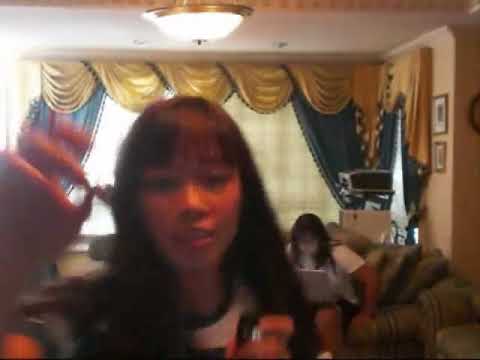The image features two women in a somewhat blurry photograph taken in a living room. The woman in the foreground is partially off-center to the left, with long dark hair and bangs. She is closer to the camera, with her left hand raised near her face, which is illuminated by a white glare, noticeable on her nose and cheek. She appears to be glancing at something, possibly a cell phone. Behind her left shoulder, another woman is seated on a green or brown couch, wearing a white shirt and focused on a laptop. Her face is barely visible due to the blurriness.

The living room is decorated with tan walls and a large window adorned with gold and blue scalloped curtains. A ceiling light fixture can be seen at the top of the image, casting light over the scene. In the background, there's a hint of electronic equipment, possibly a projector or television, and some framed pictures or paintings on the pinkish-beige walls.